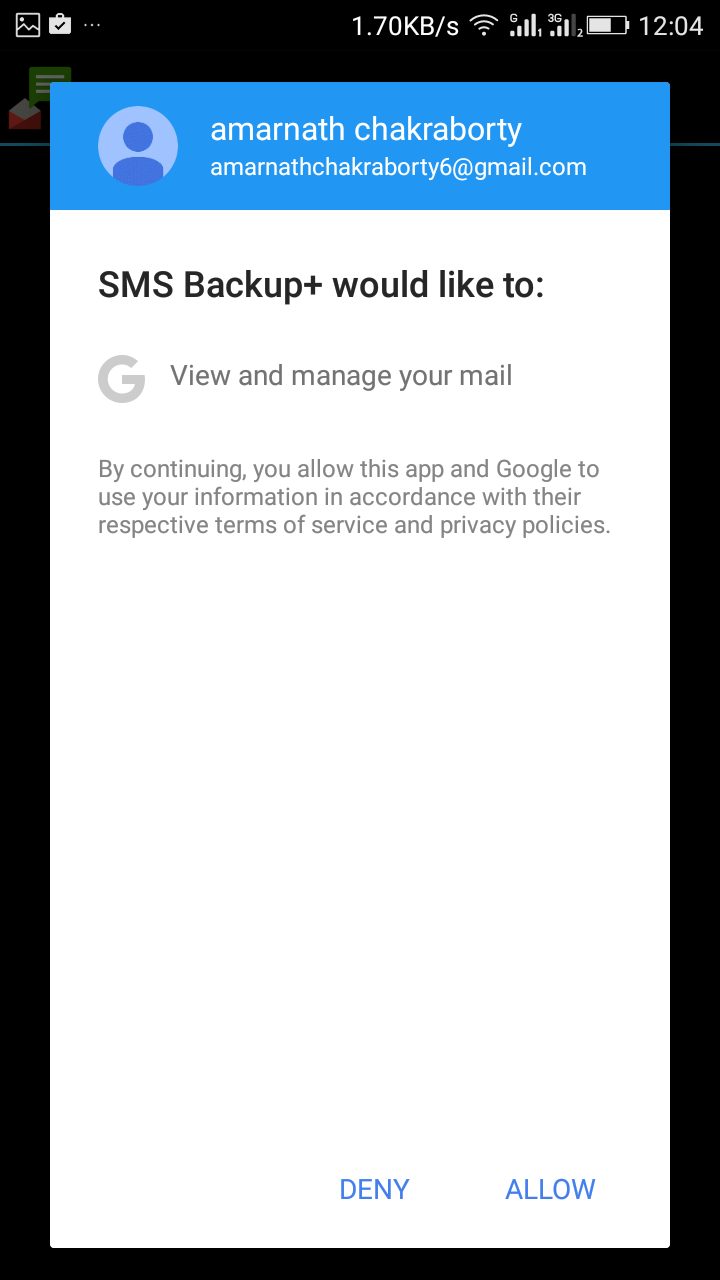The screenshot captures a mobile device screen displaying an image of a shopping bag in the top left corner. The status bar indicates a connection at 1.7 KB/s with full Wi-Fi and signal strength, while the battery icon shows almost full charge. The time displayed is 12:04. Various app icons are present, including a camera and Gmail.

A notification window occupies the center, with a white background featuring Google's 'G' logo prominently. It contains a message advising the user to view and manage their mail, with options to 'Deny' or 'Allow'. The message details that by continuing, the user agrees to the app and Google's user information requirements and transactional service policies. The screen further shows a second notification about purchasing an SMS Backup+ application for Lite 2.

The backdrop of the screen is predominantly black, highlighting the contrast with the notification windows and status bar details.